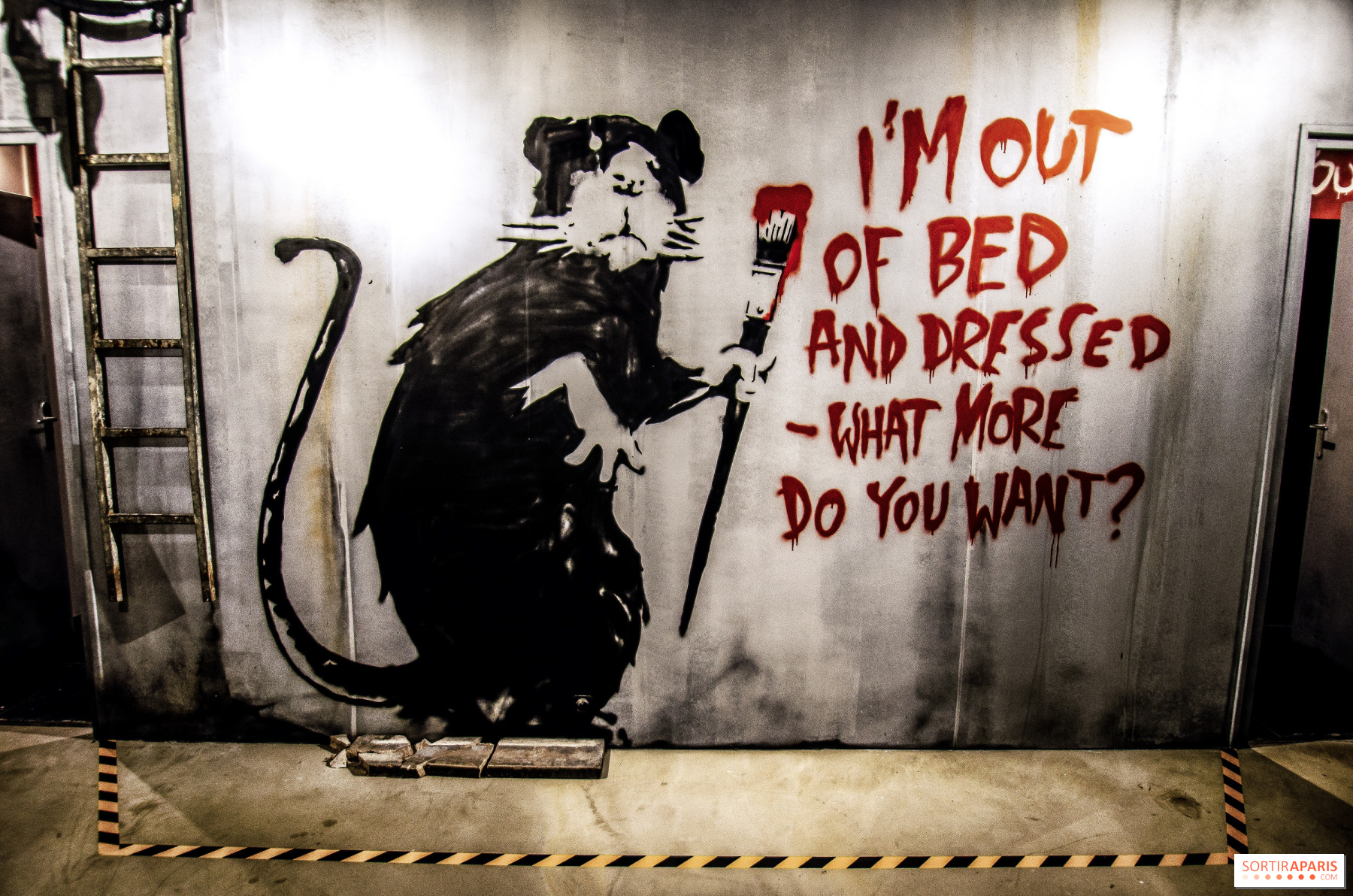The image depicts an industrial white-gray streaked wall adorned with intricate graffiti artwork, reminiscent of Banksy's style. The focal point of the graffiti is a large black rat standing upright on two feet, with a curved tail reminiscent of a coffee mug handle to the left. The rat's face and part of its stomach are white. Clutched in its left hand is an oversized paintbrush with a black handle and red paint on its white bristles. The rat appears to have used the brush to write the satirical message, "I'm out of bed and dressed, what more do you want?" on the wall. The scene is set in an industrial environment, emphasized by the tan floor marked with black and yellow "stay out" caution symbols. To the right of the graffiti, a door stands slightly ajar, revealing a dark interior tinged with a hint of red at the top. On the left side of the image, a small ladder, whose material is indeterminate, leans against the wall and extends out of the frame. The entire composition captures a gritty yet humorous urban snapshot.